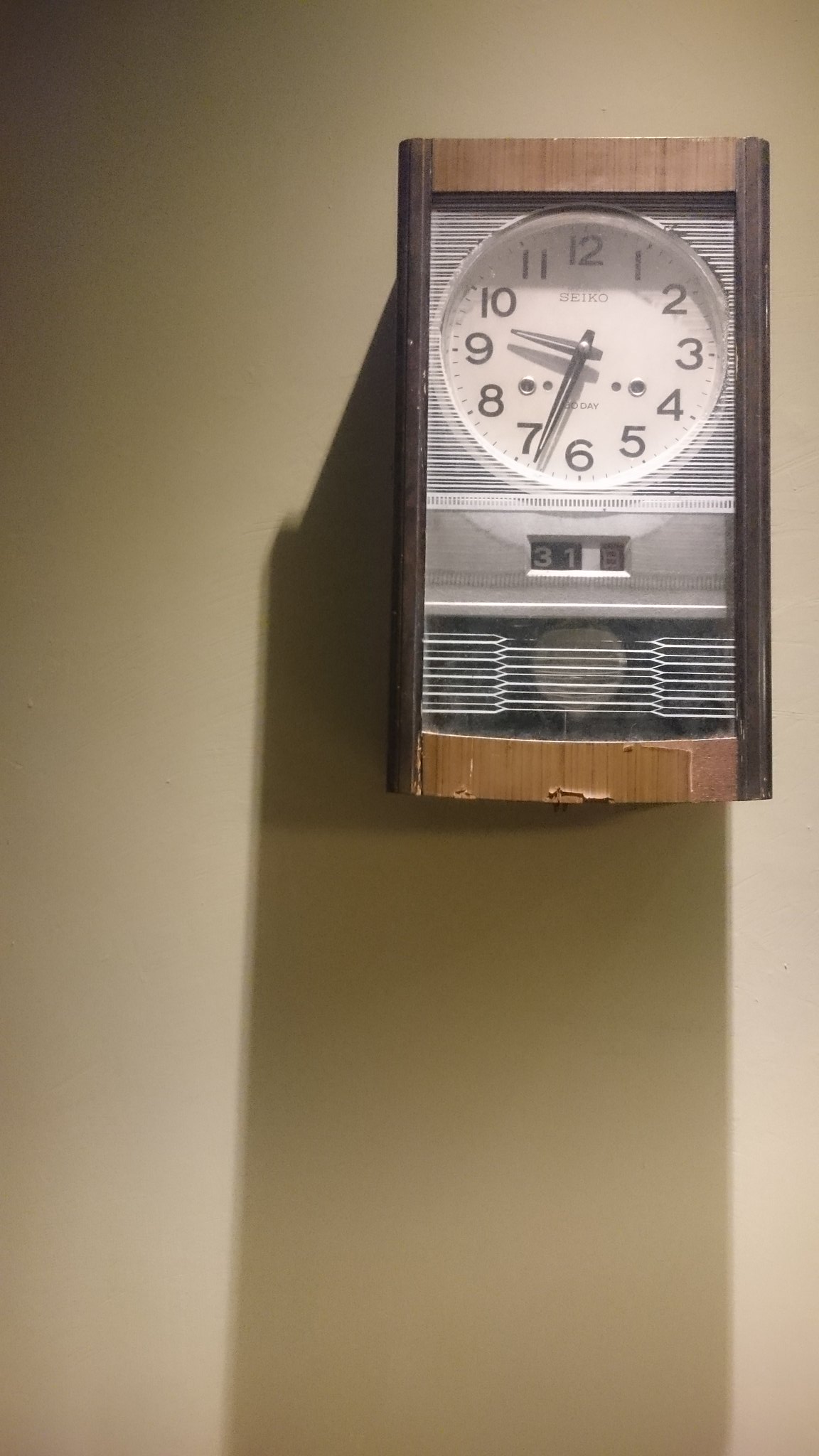A rectangular photograph captures a vintage-style wall clock mounted against a tan-colored wall. The clock features a worn wooden frame with dark wood strips on the right and left, and a medium shade wood strip at the base. Despite its antique appearance, the clock likely dates back to the 1970s or 1980s, indicated by its incorporation of both analog and digital elements. The clock's white face prominently displays large black numbers and black hands, showing the time as 9:34. The upper center of the clock face is marked with the brand name "Seiko." Just below the clock hands, the word "day" is inscribed. Further down, two cut-out sections reveal the number "31" and "8," potentially indicating the date as the 31st of August. Below this date display is a worn section that resembles a speaker, characterized by white horizontal lines over a black background. A large shadow is cast by the clock onto the wall beneath it, suggesting that an overhead light source is shining down on the scene.